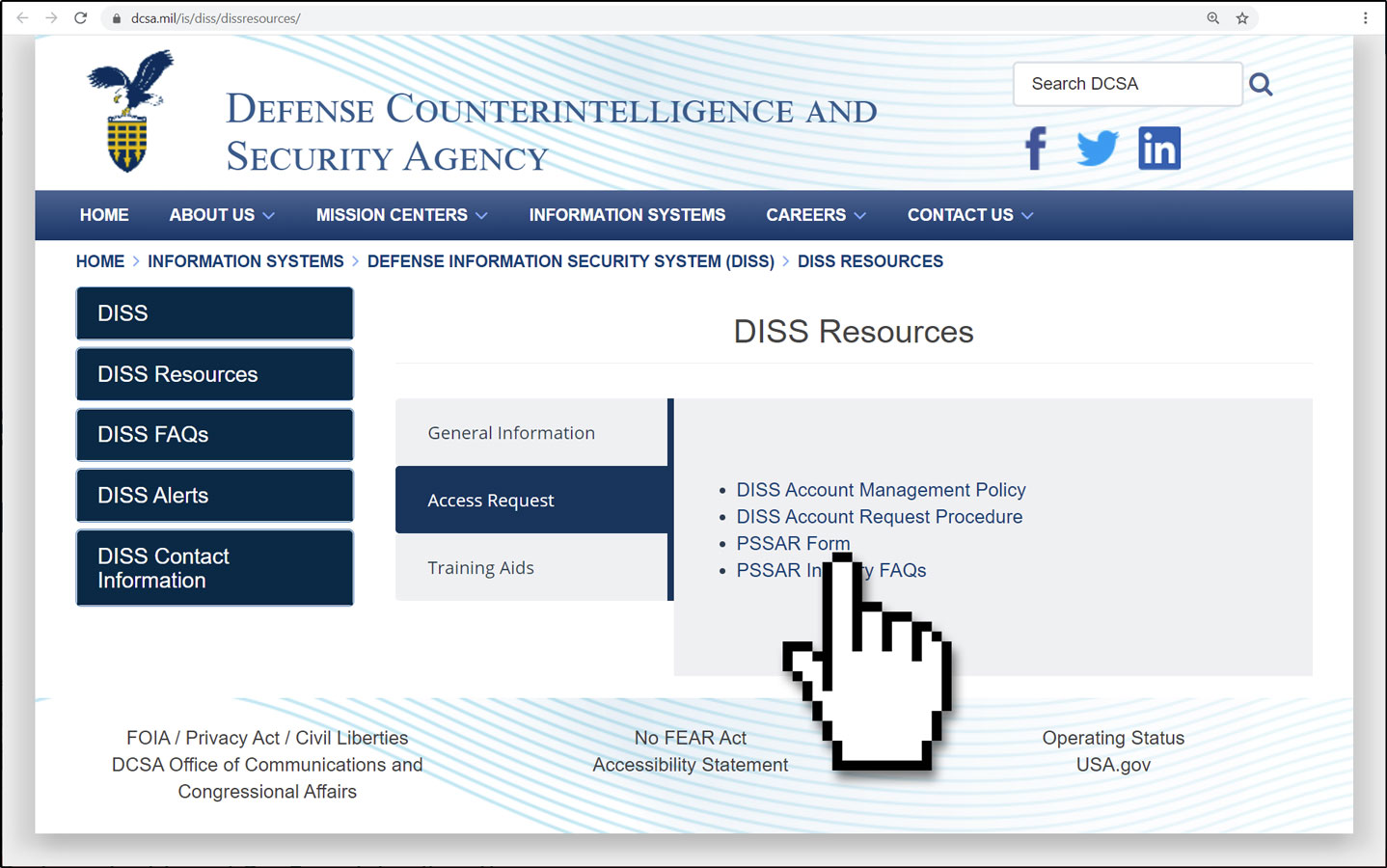**Detailed Caption:**

This image is a meticulously taken screenshot of the Defense Counterintelligence and Security Agency (DCSA) website, displayed on a MacBook interface. The characteristic design elements at the top, combined with the content, unmistakably signify that it is a military website.

In the upper left corner, a striking blue bald eagle, clutching a yellow and blue shield, symbolizes the agency's official emblem. To the upper right, there is a compact search box labeled "Search DCSA," facilitating easy navigation through the site. Additionally, the interface offers quick access to social media platforms through distinct icons: a blue 'F' for Facebook, a blue bird for Twitter, and a blue 'in' for LinkedIn.

Spanning horizontally below these elements is a prominent blue menu bar, presenting several navigational options: Home, About Us, Mission Centers, Information Systems, Careers, and Contact Us. In this screenshot, the 'Home' button is highlighted, indicating the user's current selection. 

The main content section is focused on the 'Defense Security Information System (DISS)' with a breakdown of categories such as 'Home,' 'Information Systems,' 'DISS,' and 'DISS Resources.' The emphasis is on the 'DISS Resources' section, inferred from the highlighted button. A sidebar on the left presents more specific options: DISS, DISS Resources, DISS FAQs, DISS Alerts, and DISS Contact Information. The selected sub-category 'Access Request' features a prominent large icon of a pointing finger, directing to the "PSSAR form." 

At the bottom of the screen, a footer menu provides additional informational links including the FOIA Privacy Act, Civil Liberties, DCSA Office of Communications and Congressional Affairs, the No Fear Act, Accessibility Statement, Operating Status, and USA.gov.

Given the highlighted sections and certain terms like 'DISS' and 'PSSAR form,' this screenshot might have been captured humorously or as a meme, playing on the names' amusing sound-alikes in English. This subtle layer of wordplay adds a humorous twist to the otherwise formal presentation.